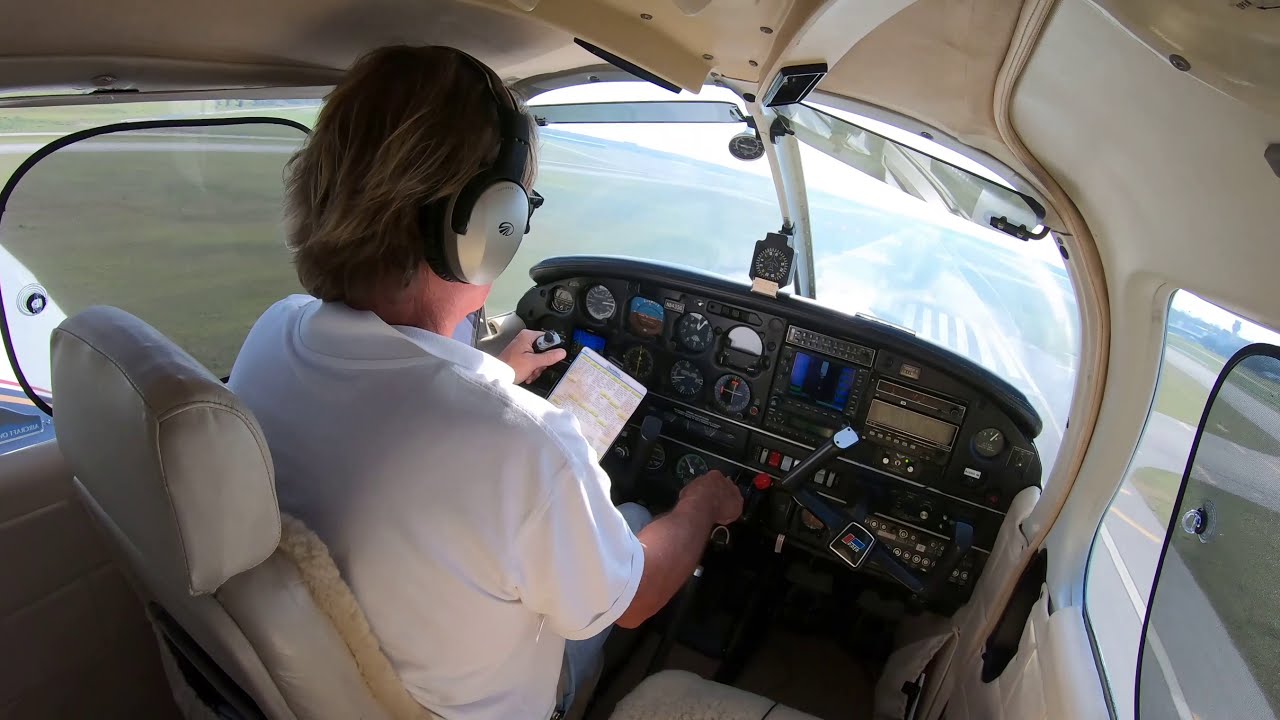In this detailed and comprehensive image description, we see a man piloting a small propeller aircraft. The photo is taken from behind the pilot, providing a clear view of the plane's cockpit and controls. The pilot, identifiable by his short blonde-brown hair, is wearing a pair of large, padded headsets and is dressed in a white polo shirt and blue jeans. Both of his hands are firmly on the control yoke as he refers to a pamphlet.

The interior of the cockpit is predominantly a light beige color, featuring an array of dials, meters, and buttons. The seats, complete with cushions, are also beige, indicating a typical two-passenger layout. Outside the cockpit, through the clear windshield and side windows, the runway is visible. It is a sunny day, and the aircraft is positioned on the runway, seemingly preparing for takeoff or landing.

To the left side of the scene, the expanse of the runway is bordered by several green grass fields. These fields suggest that the plane is at an airport, which could be either a private or international facility, given the layout. The colors in the image are various shades of white, beige, blue, brown, red, yellow, and green, capturing the vibrant and detailed environment of a sunny day at the airport.